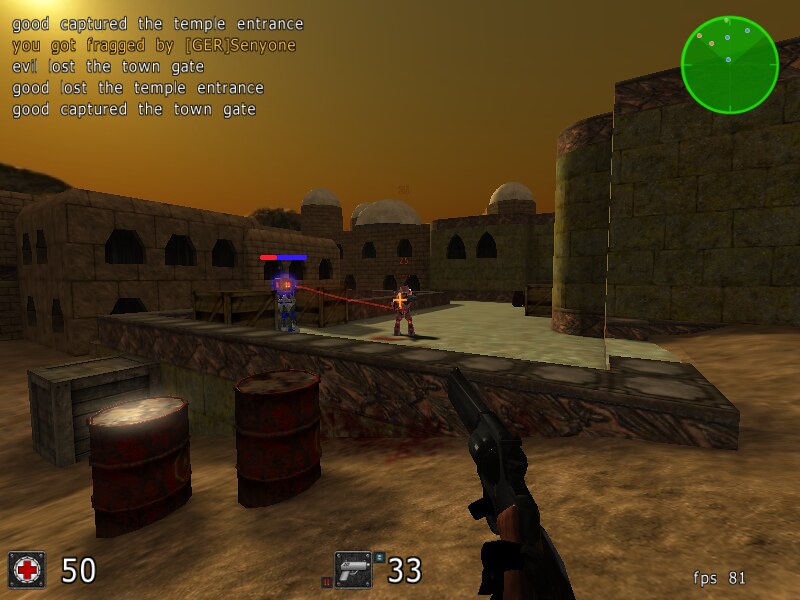The image depicts a scene from a first-person shooter video game, set in a castle-like environment with tall buildings. In the foreground, a character is aiming a gun, as indicated by the crosshair icon marked with a red "50." The gun itself displays an ammunition count of "33." In the top-right corner, the frame rate is shown as "FPS 81."

The scene is marked by numerous blood stains, hinting at recent or ongoing combat. In the distance, another character is visible, distinguished by an arrow pointing to its eyes, perhaps indicating a target or point of interest.

A minimap in the lower corner of the screen features both blue and red dots, representing different players or objectives. Text in the top corner provides a dynamic update of the ongoing objectives and statuses in the game, including instructions to "go to capture the temple entrance." Additional status updates read: "You get dragged by Jer Senon," "Evil lost the town gate," "Good lost the temple entrance," and "Good captured the town gate," summarizing recent events and current objectives within the game.